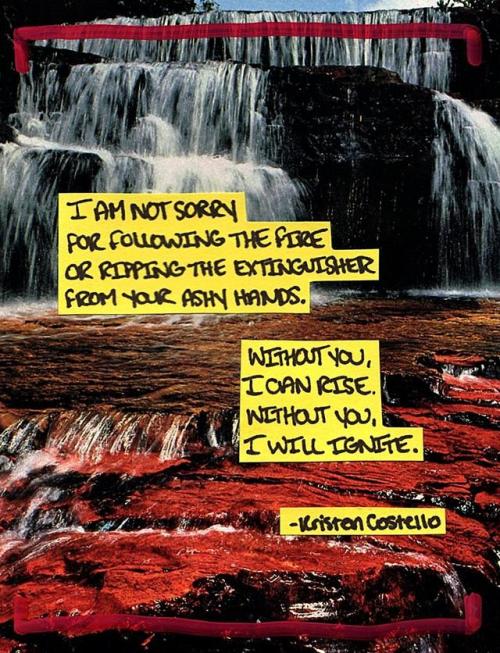The image appears to be a motivational poster or a slide from a PowerPoint presentation. It features a picturesque waterfall cascading down multiple tiers of dark, reddish-black rocks, with a river flowing towards the viewer and rippling across the foreground. A faint red line is drawn across the top of the waterfall, slightly dipping in the middle. 

In the center of the image, prominent yellow blocks of text stand out against the natural backdrop. These blocks contain black uppercase handwriting and convey a powerful message:

"I am not sorry for following the fire or ripping the extinguisher from your ashy hands.
Without you, I can rise. Without you, I will ignite."

The quote is signed with the name Kristen Costello. The white, foamy rapids of the waterfall give a sense of movement and energy, while the vivid imagery and stark contrast of colors emphasize the intensity of the message.